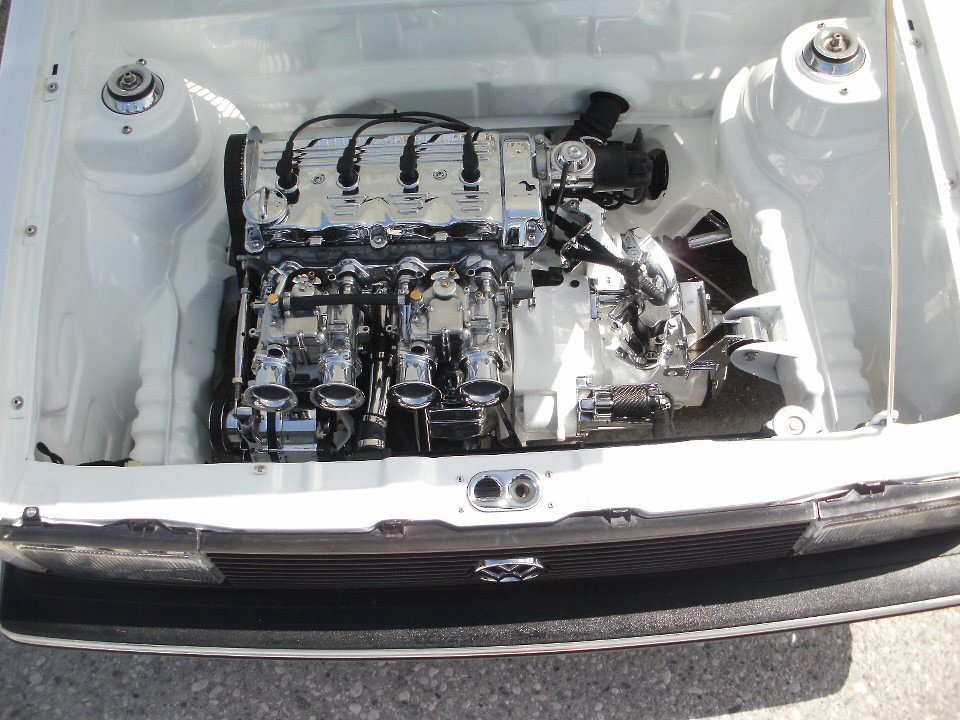This top-down digital photo showcases the clean, white interior of a Volkswagen engine bay. The ground below is a sunlit, grayish pavement with visible stones, and the shadow of the vehicle contrasts with the bright driveway. The focal point is the sparkling silver motor, surrounded by a white trim along the edges. The engine, which appears to sit lower down in the compartment, features several black components and four black ignition cables extending from a large silver section. There's a light brown stick holding up the hood. Notable details within the engine bay include two round metal spheres on the left and right, along with a prominent black grille at the front adorned with the iconic Volkswagen logo. Situated on either side of the grille are two clear headlights, contributing to the meticulous and polished appearance of the vehicle.